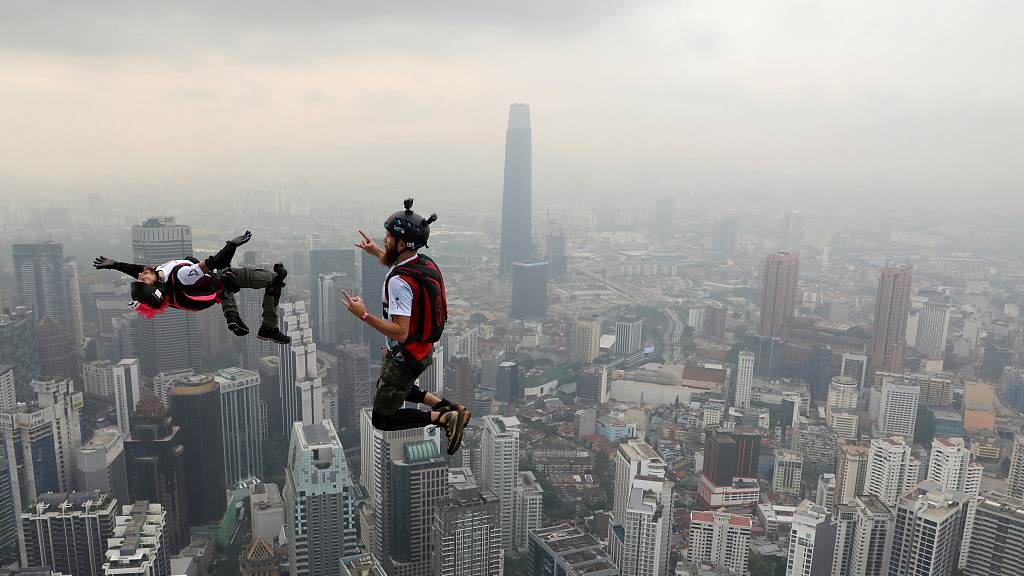In this detailed photograph taken in an outdoor setting, we see two skydivers suspended in mid-air. They are equipped with black helmets, GoPro cameras, safety gear, and parachutes that remain unopened on their backs. One skydiver lies horizontally with arms spread wide, while the other is in a semi-kneeling position with hands visible. Both individuals, who appear Caucasian, are dressed in a combination of red, black, and white outfits.

The background reveals an extensive urban cityscape below them, featuring numerous skyscrapers and other tall buildings, typical of a major metropolitan area. Notably, there is one exceptionally tall building that stands out in the center-right of the image. The sky above the city is predominantly grayish and light brown, with varying shades of grey clouds, including a particularly dark patch in the top left corner. A hint of pink breaks through the fog and smog, giving the sky a somewhat polluted appearance. The image captures the breathtaking, albeit smoggy, aerial perspective of the two skydivers soaring high above the bustling city below.